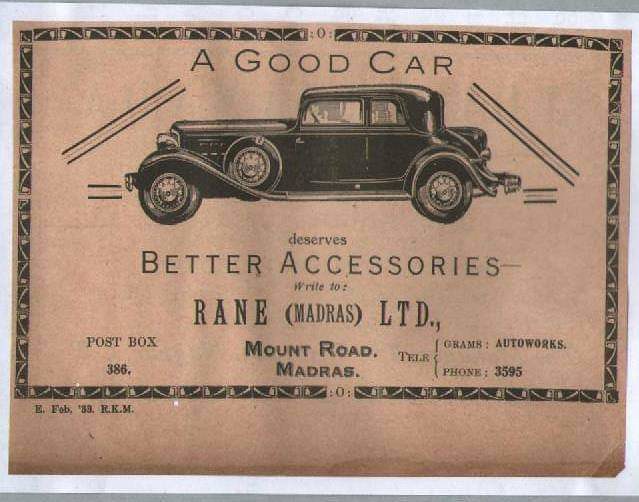The image is an aged, rectangular advertisement that appears to have been cut from a newspaper, characterized by a white border framing a beige, parchment-like background. An intricate rectangular border adorns this paper, giving it an elaborate and old-time feel. At the very top, in bold black lettering, the text reads "A Good Car," followed by an illustration of an old-fashioned Ford from the early 1900s, depicted in a side view with a spare tire on its side, facing left. Below the car, the caption continues with the phrase "deserves better accessories" in the same black lettering. 

This advertisement promotes Rain Madras Limited, providing their contact details: Post Box 386, Mount Road, Madras. To the lower right of the text, their phone number is also listed. Additional small print outside the main framing mentions "EFEB" and possibly "53 RKM" or "KKM," though this part is difficult to decipher. The overall appearance hints at its historical context, likely from the 1950s or 1960s, emphasizing the period's style and the advertisement's focus on enhancing car accessories.